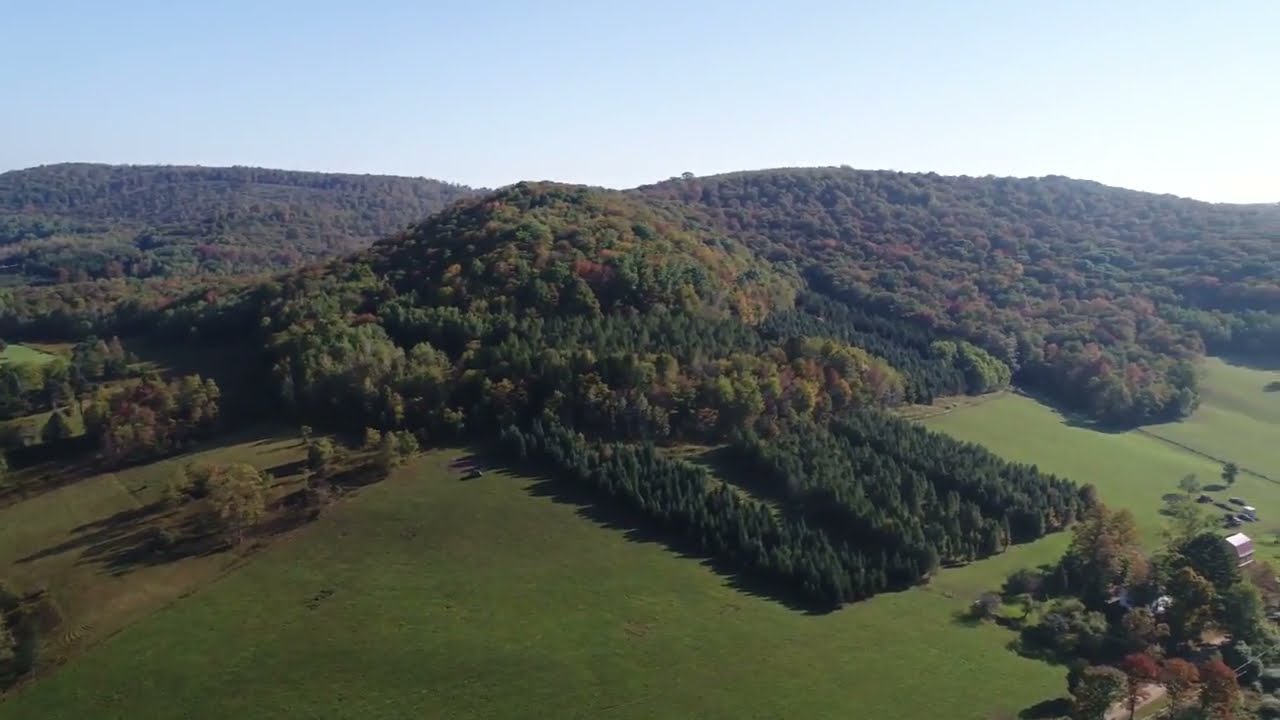This detailed aerial color photograph captures a vibrant expanse of natural landscape dominated by various shades of green, with touches of brown and reddish hues. The scene is one of unspoiled wilderness, showcasing a large grass field surrounded by dense clusters of trees, depicting a serene, undisturbed outdoor environment bathed in natural daylight. The top portion of the image features a bright blue sky, gradually lightening towards the right, providing a clear, bright backdrop that enhances the clarity of the overall image. 

The photograph reveals a terrain marked by rolling hills and valleys, adding depth and dimension to the vista. Central to the image is a prominent tree-covered mound, with a distinctive rectangular section of orderly planted dark green trees positioned slightly to the right. In the background, the landscape extends into a series of forest-covered hills and mountain ranges, contributing to the sense of vast natural beauty. 

In the bottom right corner, partially concealed by trees, is a cluster of agricultural buildings. Notably, the image does not feature any vehicles, people, or animals, maintaining its focus on the untouched, picturesque quality of the landscape. The clear and bright setting, accentuated by drone photography, lends a realistic and representational style to this evocative depiction of nature.